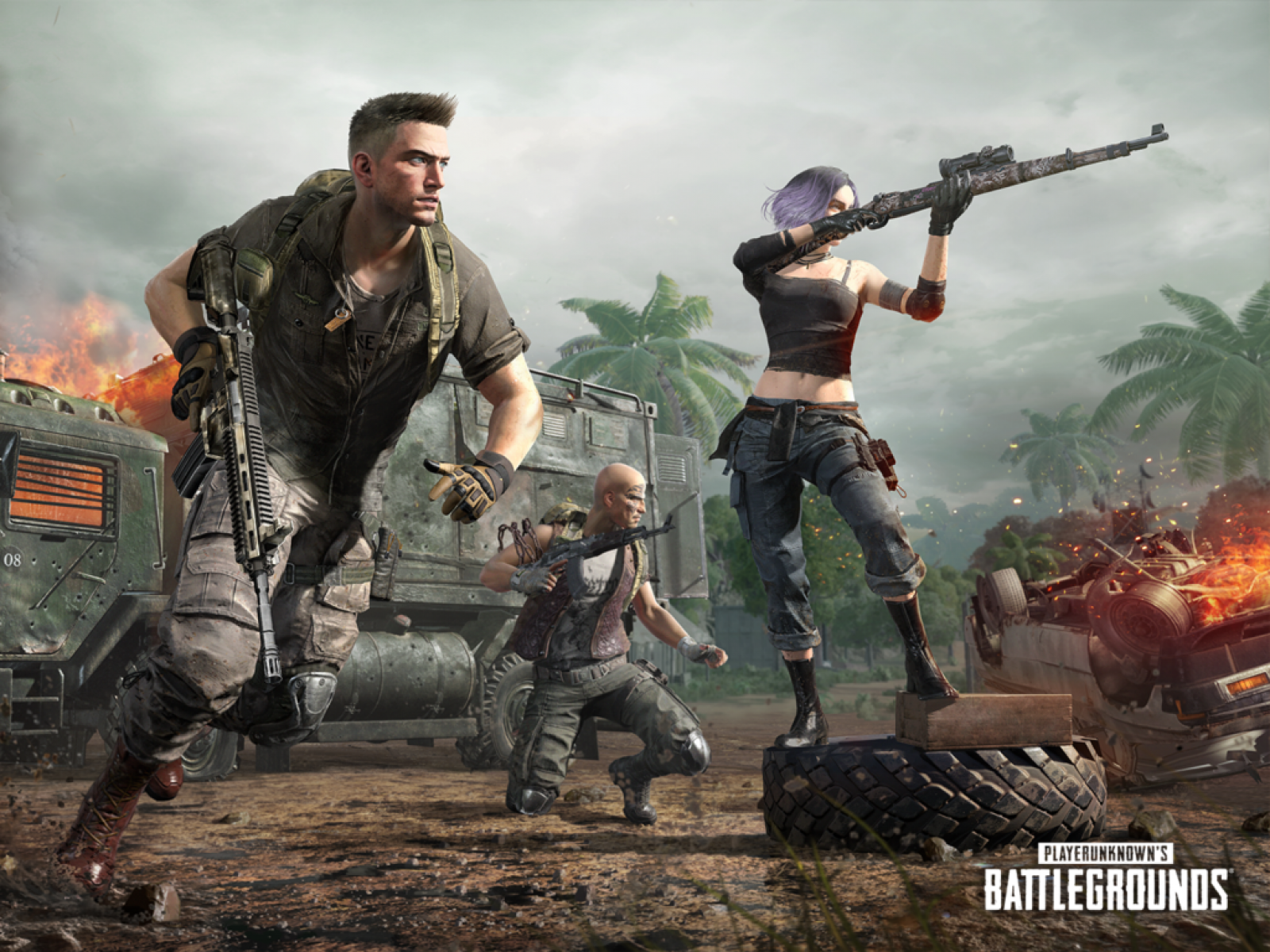The screenshot from the game PlayerUnknown's Battlegrounds depicts an intense battle scene set in an outdoor, smoky environment. The sky appears gray and hazy, contributing to the chaotic atmosphere. In the background, there is an overturned vehicle engulfed in flames. On the left side, a green military truck can be seen, reinforcing the war-torn setting. Central to the scene are three characters, all armed and moving towards the right.

One character, a woman with short light purple hair, stands prominently on top of a large tire. She is dressed in jeans, a crop top, and black boots, holding a scoped rifle aimed towards the right. Accompanying her is a man in an olive green army shirt with short sleeves, gray cargo pants, and brown boots. He carries a military bag and a machine gun, moving purposefully forward with a buzz cut. The third character is a bald man kneeling on one knee, wearing a red vest and dark gray or green cargo pants, scanning the distance with his gun raised.

Together, the trio appears to be advancing towards an unseen threat, embodying the game's high-stakes survival theme. The official PlayerUnknown's Battlegrounds logo is visible in white at the bottom of the image, anchoring it as both an advert and a glimpse into the game's immersive environment.